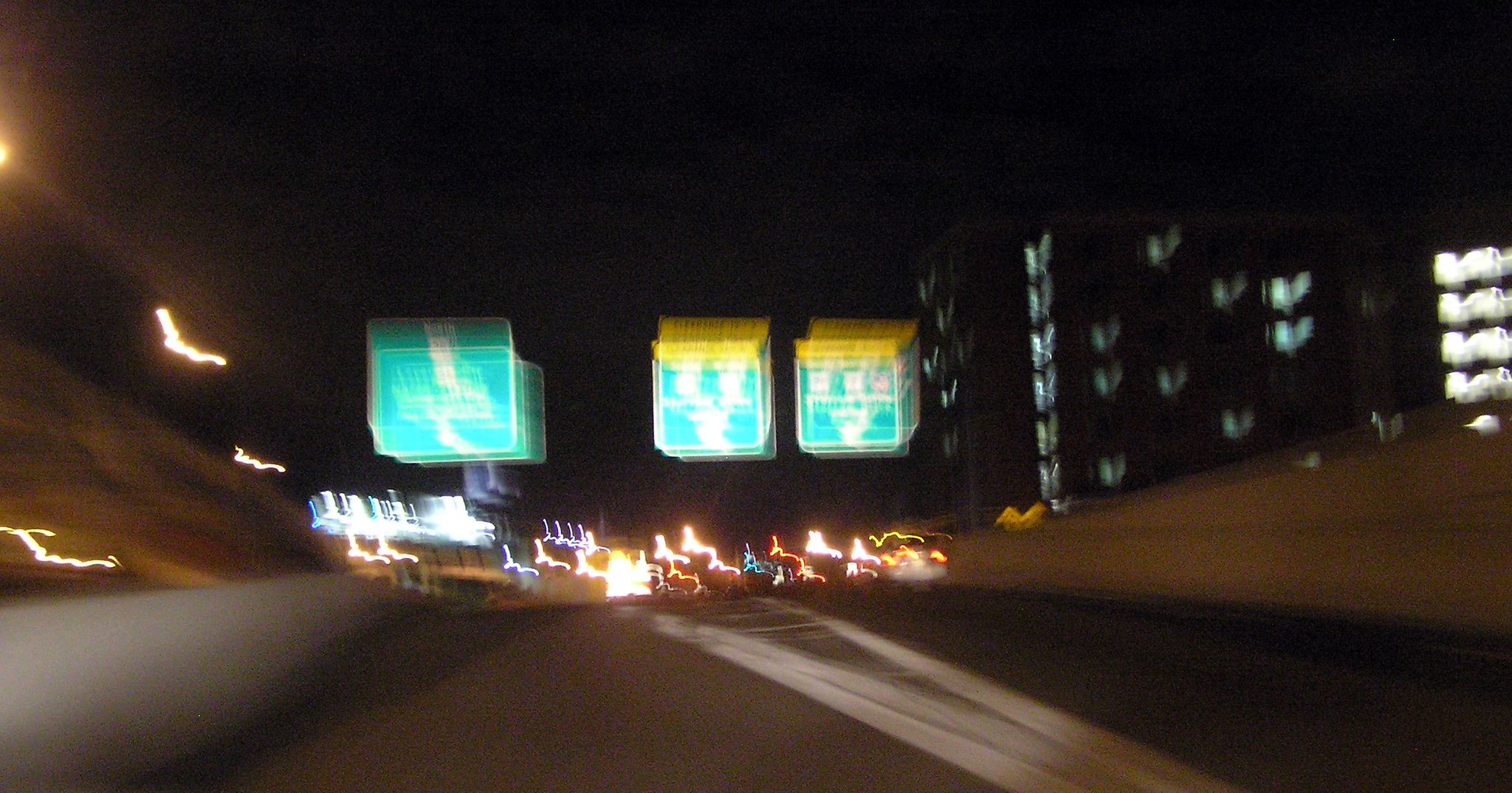The image captures a bustling highway at night, featuring three directional signs prominently displaying routes and destinations. A car is in motion, creating light trails against the dark backdrop. Streetlights cast linear glows across the scene, illuminating the road. To the left, a softly lit hill slopes upwards, adorned with bright lines likely marking pathways. On the right, a large apartment building stands tall, with numerous windows aglow, reflecting the activity within. Further to the right, an illuminated parking garage spans several floors, each level clearly visible. A distinct white V-shaped divider marks the center of the highway, guiding traffic flow under the urban night sky.